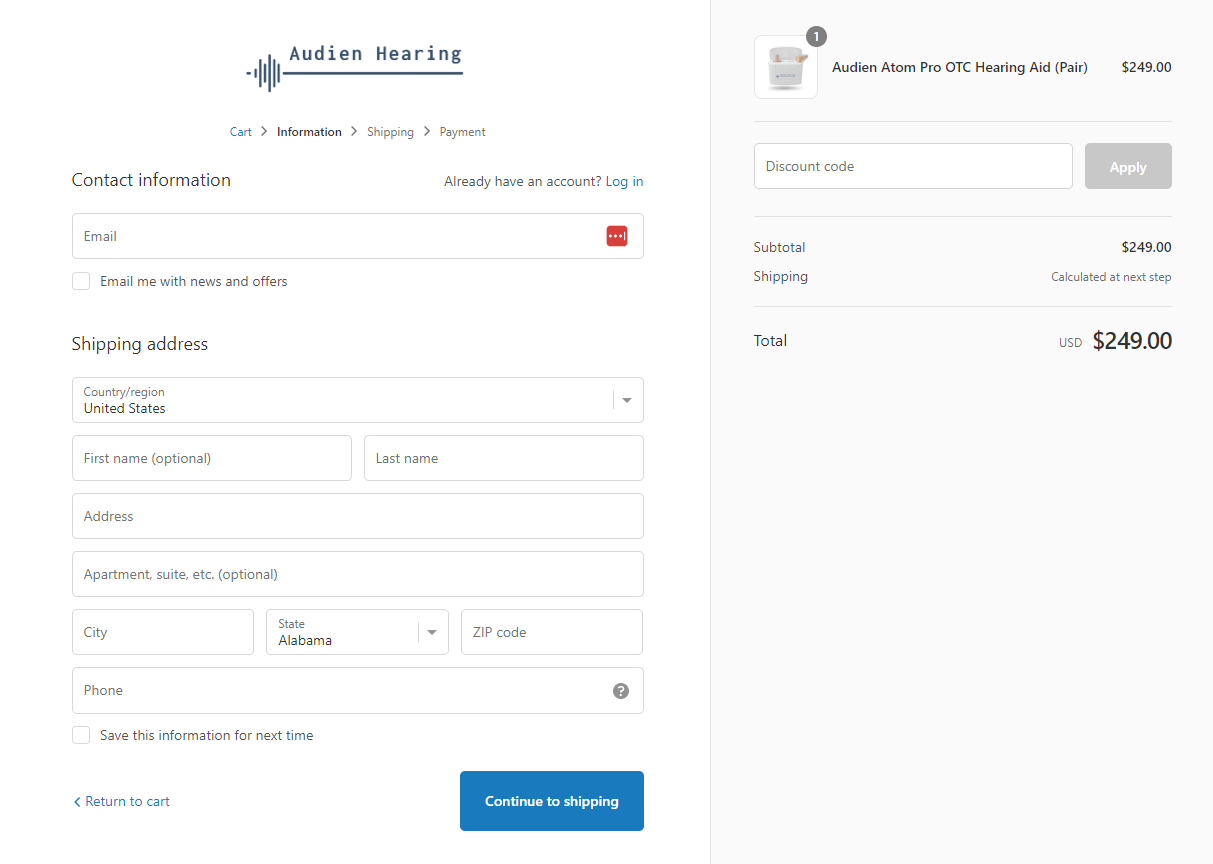The screenshot depicts two distinct sections of the AUDIEN hearing payment process.

**Left Screenshot**:
- The screen features a white background with the AUDIEN Hearing logo prominently displayed.
- Users are greeted with elements including "Cart Information," "Shipping," and "Payments," indicating that they are at the payment stage.
- There's a section for contact information with a prompt for users who already have an account to log in.
- Below that, there is an email input field with an optional checkbox to receive news and offers via email.
- The shipping address section includes input fields for country/region (dropdown menu), first name (optional), last name, address, apartment/suite (optional), state (dropdown menu), zip code, and phone number.
- Users can opt to save this information for future use by ticking a checkbox.
- Navigation options at the bottom include a "Return to Cart" button with a left arrow on the bottom left, and a "Continue to Shipping" button on the bottom right.

**Right Screenshot**:
- This section displays product details on a light gray background.
- The product highlighted is the "AUDIEN Adam Pro OTC Hearing Aid Pair" priced at $249.
- There is an input field for a discount code accompanied by an "Apply" button.
- The subtotal amounts to $249, with a note that shipping costs will be calculated at the next step.
- The total amount is listed as $249.00 USD.

Together, these screenshots provide a comprehensive view of the payment and shipping information entry process for purchasing AUDIEN hearing aids.